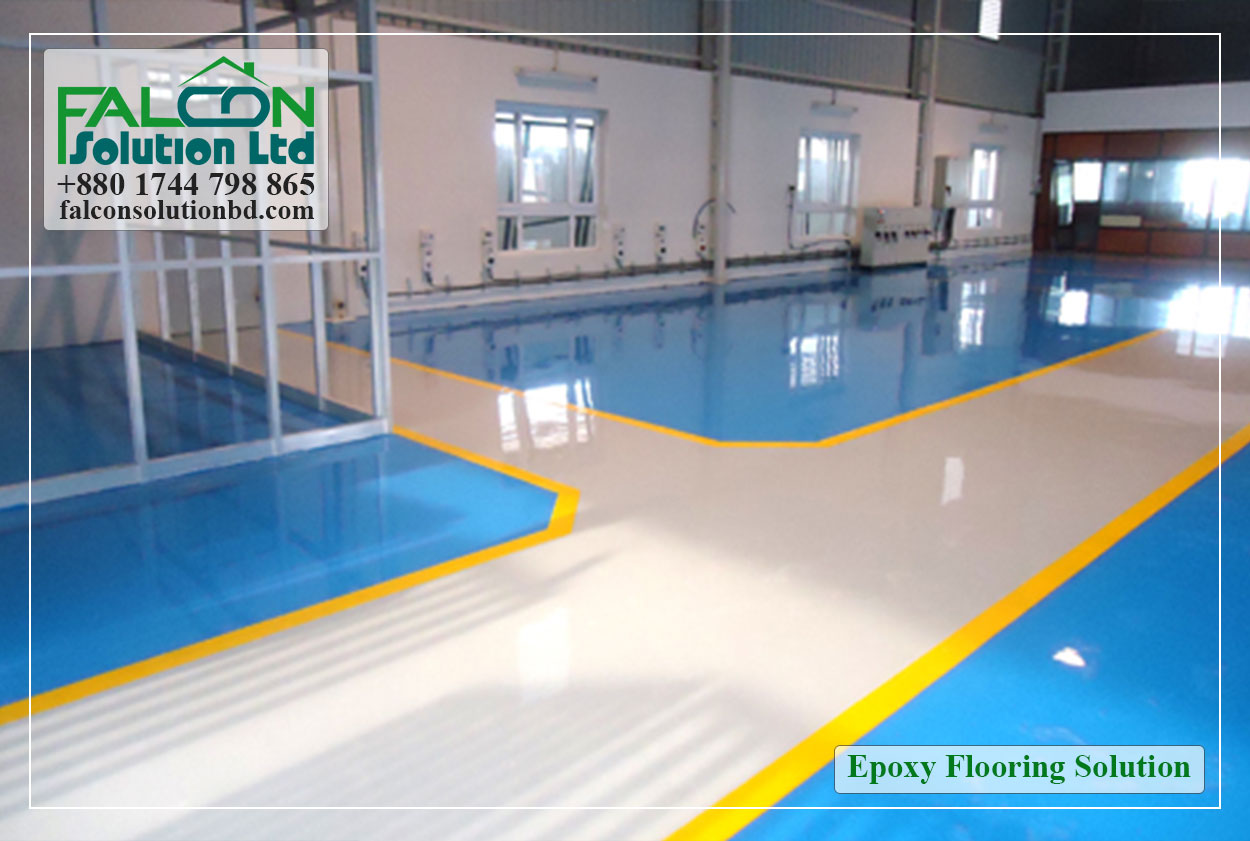The image showcases an epoxy flooring solution presented by Falcon Solution LTD. In the top left corner, there is a white square with the company's name in green, with a logo featuring a rooftop motif within the "CO" of "Falcon." Below this, their contact number, "880-1744-798865," and the website, "falconsolutionbd.com," are displayed in black text. On the bottom right, another white rectangle features the green text "Epoxy Flooring Solution."

The setting appears to be an industrial or showroom space, possibly a gymnasium or warehouse. The floor is a glossy, vibrant blue, accentuated by a cream-colored walkway edged in yellow, leading towards a door and extending to the other side of the room. The left-hand side of the image reveals a steel bar structure resembling prison bars with larger gaps. The walls are a mix of white, gray, and wooden textures, with multiple windows – three on the left wall and a long window on the forward-facing wall, framed with brown accents. Between two of the windows, some machinery is visible, adding to the industrial ambiance. The overall impression is a clean, polished, and professional space aimed to showcase the quality and aesthetics of the epoxy flooring.